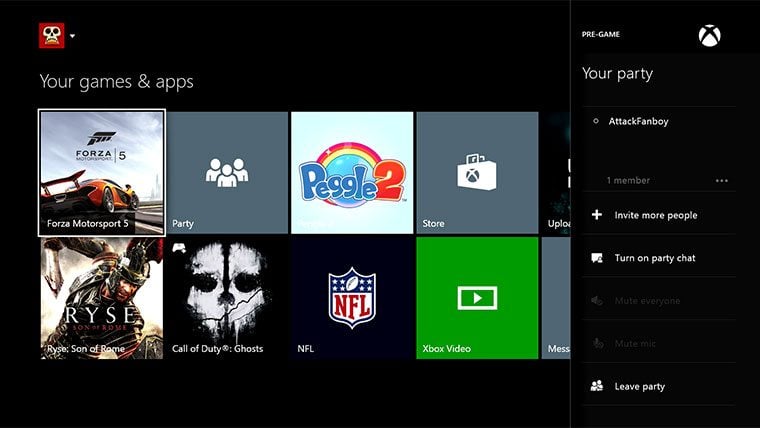In the upper left corner of the image, "Your Games & Apps" is prominently displayed. In the upper right corner, there is a red icon featuring a white skull with black eyes, nose, and mouth, accompanied by a pull-down menu. Below this header, a selection of app and game icons is arranged in two rows of four square images each. Visible titles in these rows include "Forza Motorsport 5," "Party," "Peggle 2," "Store," "Ryse," "Call of Duty: Ghosts," "NFL," and "Xbox Video." Additional icons are partially visible on the right side, both above and below these rows. 

To the right of the squares, the word "Pre-Game" appears with an Xbox symbol (a circle with an X inside) directly below it. The "Your Party" section is beneath this, listing a party named "Attack Fanboy," which currently has one member. Adjacent to this are ellipses and options including "Invite More People," "Turn On Party Chat," "Mute Everyone," "Mute Mic," and "Leave Party." The options "Mute Everyone" and "Mute Mic" are shown in a gray color, blending with the background, while the rest of the options are highlighted in white.